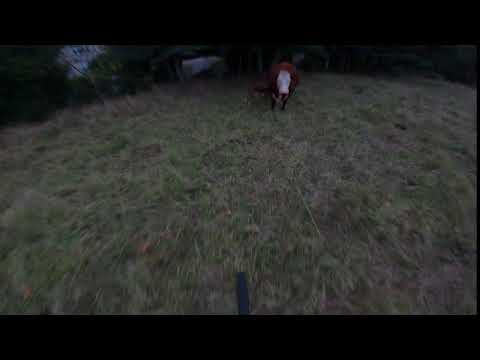The image captures a dimly lit outdoor scene dominated by a large, uneven grassy field that bears patches of brown and green. The foreground is blurry, dotted with indistinct shapes and a narrow blue rectangle. A clear black border frames the top and bottom of the image, adding to its overall dark tone. In the distance, within the middle of the image, there's a figure—possibly a person wearing a red and white outfit with their legs faintly visible—standing amidst a scattered arrangement that could be bushes or trees. Impressions of lighter objects, potentially glimpses of the sky or buildings, peek through the dense foliage stretching across the background. Despite the pervasive darkness, the faint details suggest an outdoor setting filled with natural elements.